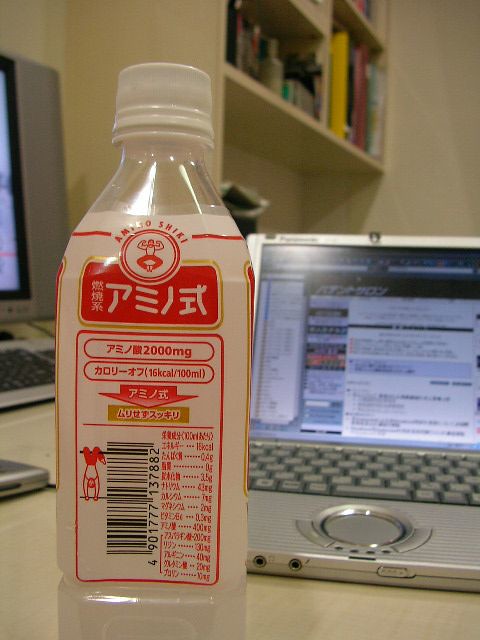The image depicts a small, square, clear plastic bottle containing a cloudy white beverage with primarily Japanese text on its label, including the transliterated word "AMINO SHIKI" at the top in red within a rectangle. The bottle features a white cap and a white plastic label that wraps around its bottom half. The larger vertical red outline on the label includes the number "2000mg," followed by more Japanese text and a downward arrow. Below the arrow, additional numbers such as "16kcal/100ml" are noted. A cartoon image of a man flexing his muscles is also present. A large central barcode (4901777137882) and a nutritional panel oriented vertically on the right side are visible on the label. The bottle is positioned on a white table. In the background, an open silver laptop with a dark gray keyboard is discernible. To the far left, a desktop computer screen is part of the scene. Above the table, the upper area of the photo shows a built-in bookshelf with various colored books and binders.